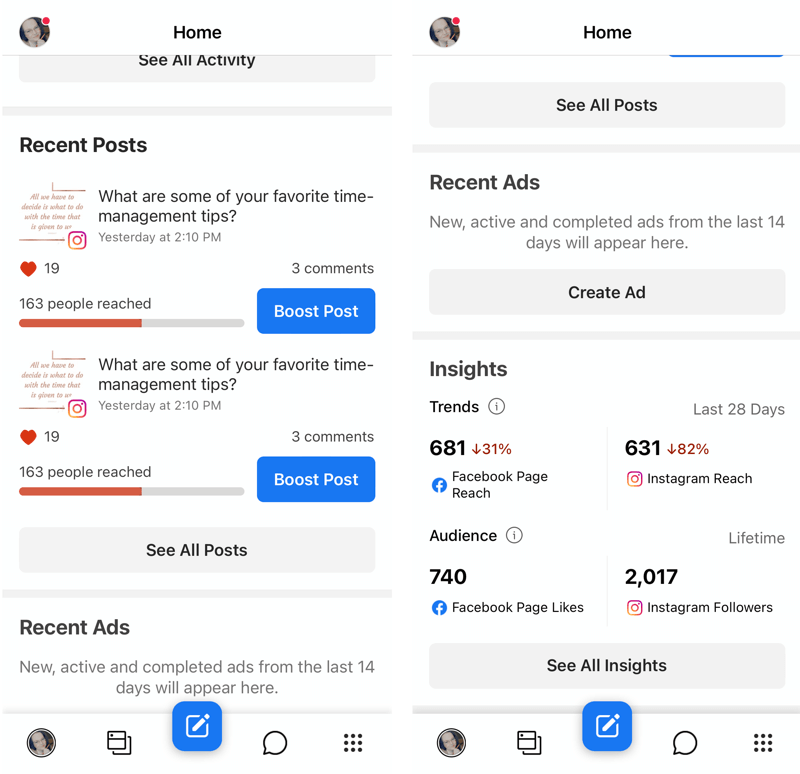In the upper left corner of the image, there is a circular profile picture showing a person with dark hair, glasses, and white skin. Adjacent to this profile picture is a red circle, and below it is the word "Home." Beneath this, there is a section titled "See All Activity" followed by "Recent Posts." Under "Recent Posts," a question reads, "What are some of your favorite time management tips?"

Towards the middle of the image, there is a small pink square icon representing Instagram, featuring a pink circle inside it. Next to this icon is a heart symbol with the number 19 beside it, indicating interactions, and the text "163 people reached" with a red bar below it. Adjacent to this red bar is a blue rectangle with the text "Boost Post" inside it.

On the right side of the image, there is an option labeled "See All Posts," followed by "Recent Ads." This section mentions that new, active, and completed ads from the last 14 days will appear there and features an option to click "Create Ad" inside a gray rectangle.

Below this, there is a section called "Insights," under which the word "Trends" is displayed. Next to "Trends" is the number 681 accompanied by a red arrow pointing downward, indicating a 31% decrease. Further below, there is a section labeled "Facebook Reach" featuring the Facebook emblem, a lowercase "f" inside a blue circle. To the right of this is the number 631 with a red arrow pointing downward, indicating an 82% decrease. Lastly, there is an "Instagram Reach" section with the Instagram pink square icon mentioned earlier.